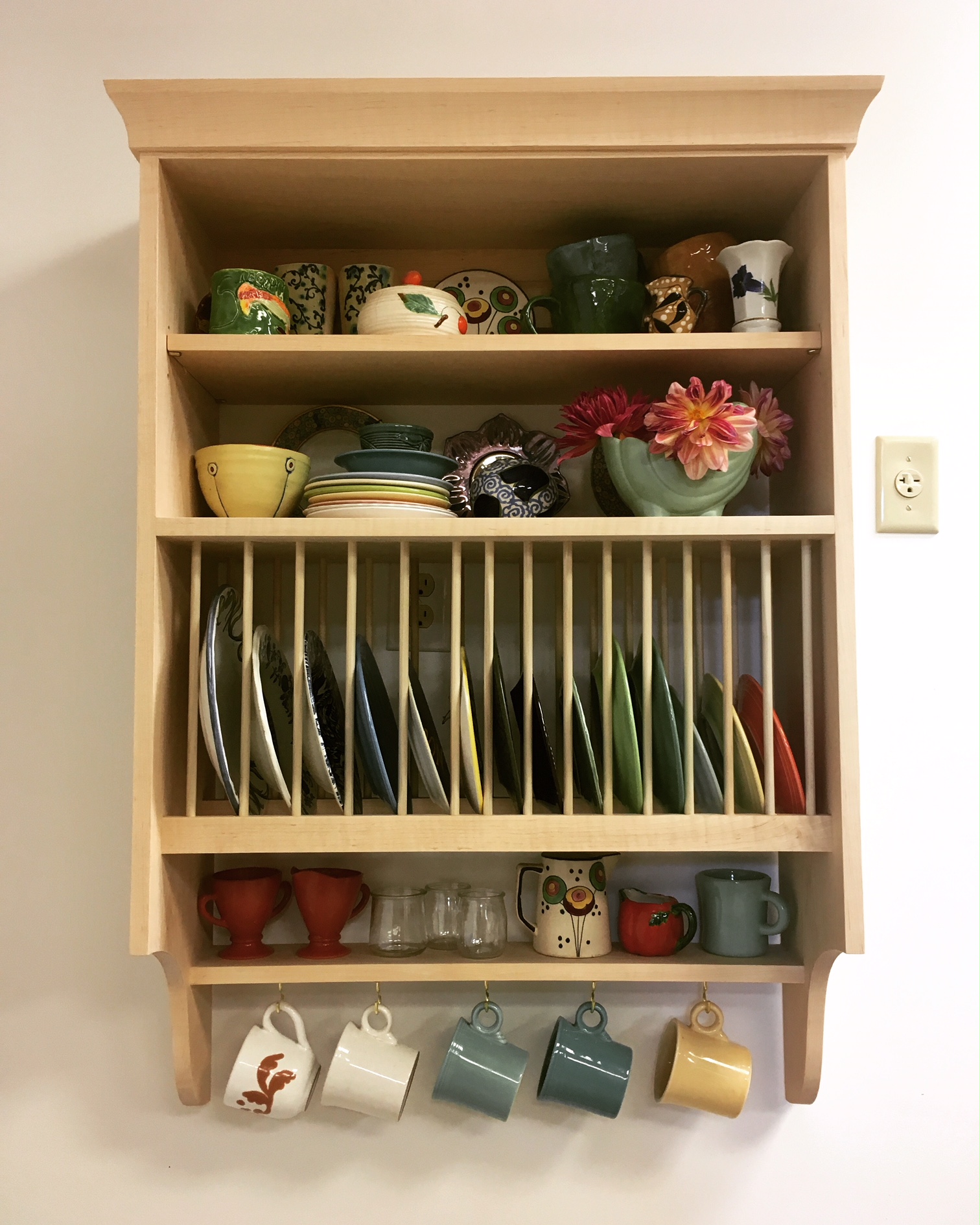A meticulously organized wooden kitchen cabinet is displayed in the image, showcasing a variety of dishware and cups. The cabinet is crafted from rich brown wood, adding a warm, rustic charm to the kitchen. On the topmost shelf, an array of colorful teacups is neatly arranged, creating a vibrant focal point. The middle shelf holds a collection of plates and a decorative arrangement of flowers, adding a touch of elegance. Individual compartments on another shelf host an assortment of cups, enhancing the orderly appearance. Finally, the bottom section features five hanging cups in green, white, and yellow hues, adding a whimsical touch to the practical storage solution. This well-crafted cabinet not only serves as a functional kitchen element but also as an aesthetically pleasing display of everyday dishware.